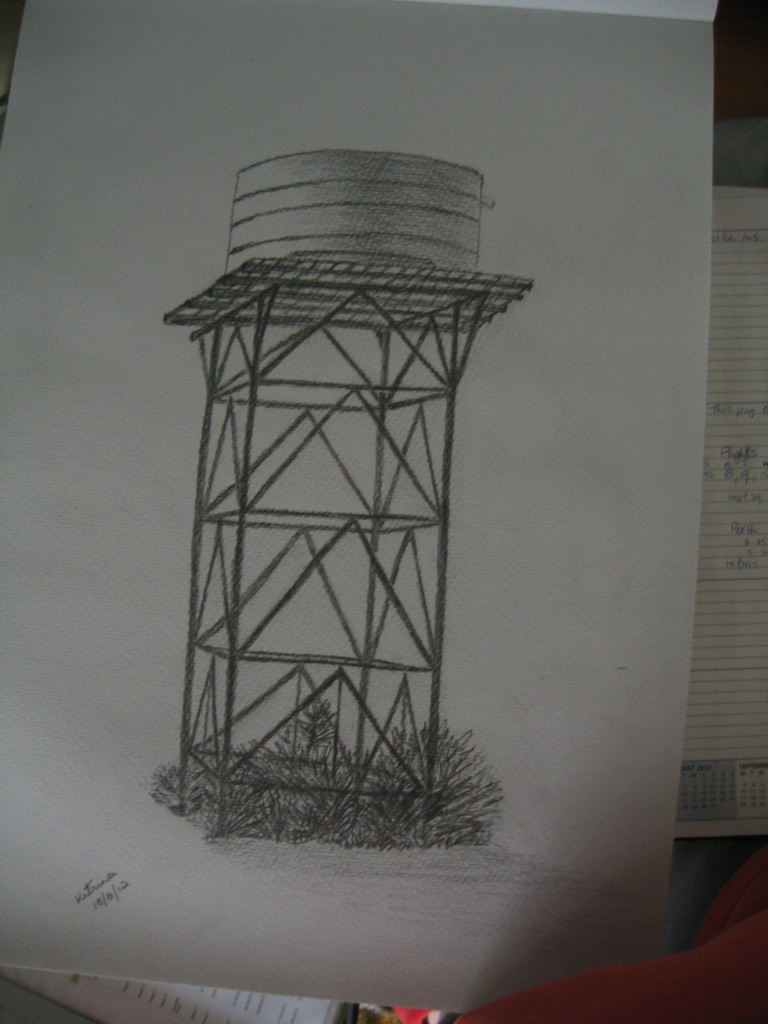A meticulously detailed sketch, rendered in dark pencil on a large white sheet of paper, captures a water tower with intricate precision. The water tower features a substantial frame supporting a flat-topped platform, crowned by a cylindrical tank with an outward protrusion on its side. Verdant plants flourish beneath the structure, their foliage delicately illustrated, while subtle shading accentuates the ground surrounding the tower. Though the artist’s signature and date are visible at the bottom left, they remain too small to decipher. The scene is set within an interior space, evidenced by a lined notebook with blue ink writing and several other books or miscellaneous objects scattered at the bottom of the photograph. A hint of red cloth at the edge suggests the presence of the photographer, possibly part of their attire.